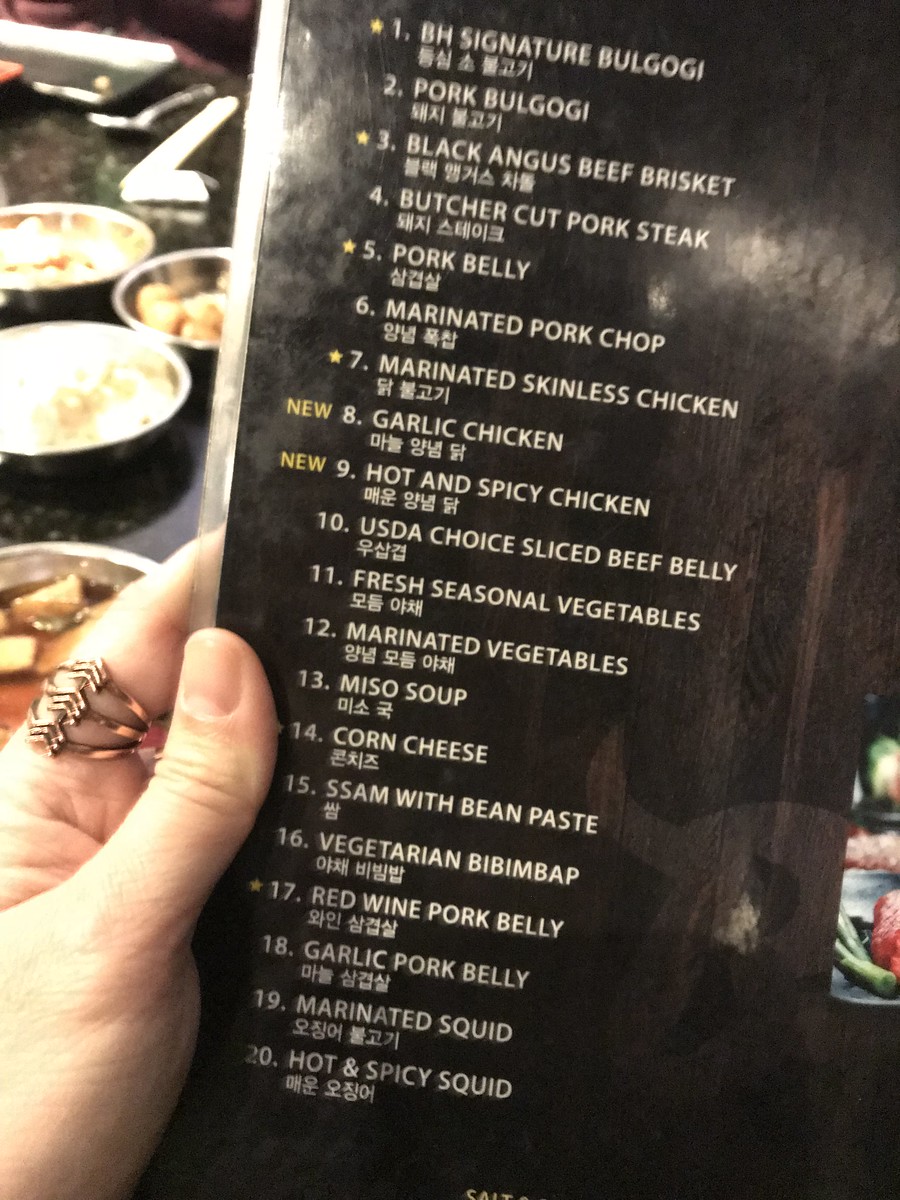The photograph features a menu being held by a slender white hand, believed to belong to a woman. She is wearing a gold-tone, three-section ring on her pointer finger, positioned near the base. In the left part of the image, there are several plates, including a bowl of mashed potatoes and a couple of other bowls with unidentifiable contents. The menu lists various dishes with corresponding Asian writing, detailed as follows:

1. BH Signature Bulgogi
2. Pork Bulgogi
3. Black Angus Beef Brisket
4. Butcher Cut Pork Steak
5. Pork Belly
6. Marinated Pork Chop
7. Marinated Skinless Chicken
8. New: Garlic Chicken
9. New: Hot and Spicy Chicken
10. USDA Sliced Beef Belly
11. Fresh Seasonal Vegetables
12. Marinated Vegetables
13. Miso Soup
14. Corn Cheese
15. Ssam with Bean Paste
16. Vegetarian Bibimbap
17. Red Wine Pork Belly
18. Garlic Pork Belly
19. Marinated Squid
20. Hot and Spicy Squid

To the right of the menu, there is a small plate containing some fresh produce.